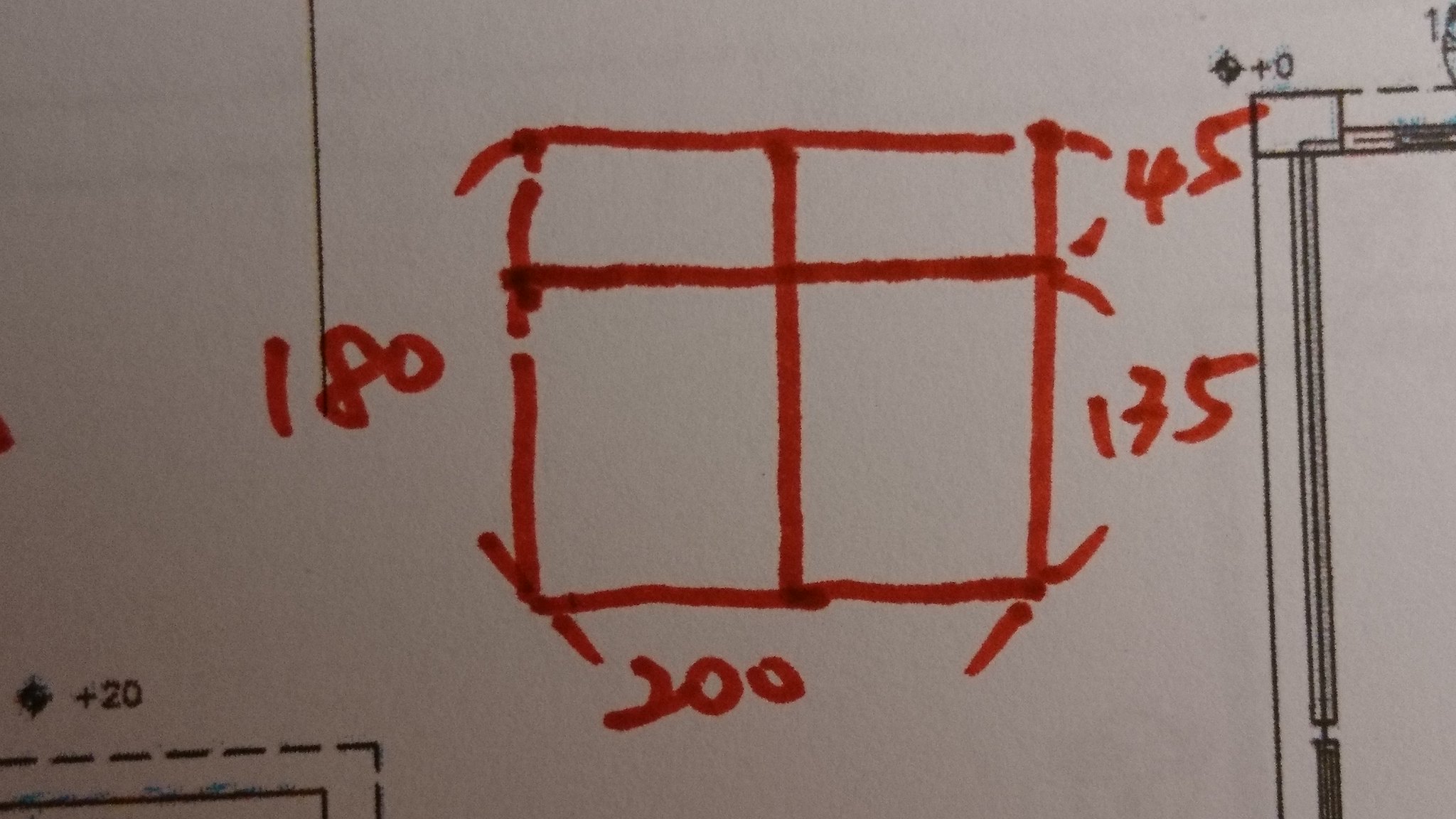The photograph depicts a section of a drafting document adorned with both printed lines and numbers in black, alongside handwritten notes in red magic marker. Central to the document is a meticulously outlined box, subdivided into four rectangles—two narrow ones at the top and two taller ones at the bottom. Marked within this hand-drawn boundary are precise numerical annotations: ‘45’ at the upper right, ‘135’ at the lower right, ‘200’ at the bottom, and ‘180’ on the left side. Extending from each corner of the box are additional lines: one each at angles from the bottom left and bottom right corners, and one each from the upper left and upper right corners. This blend of detailed penmanship and technical precision suggests the document is part of a larger architectural or engineering draft, capturing both measured accuracy and purposeful annotation.